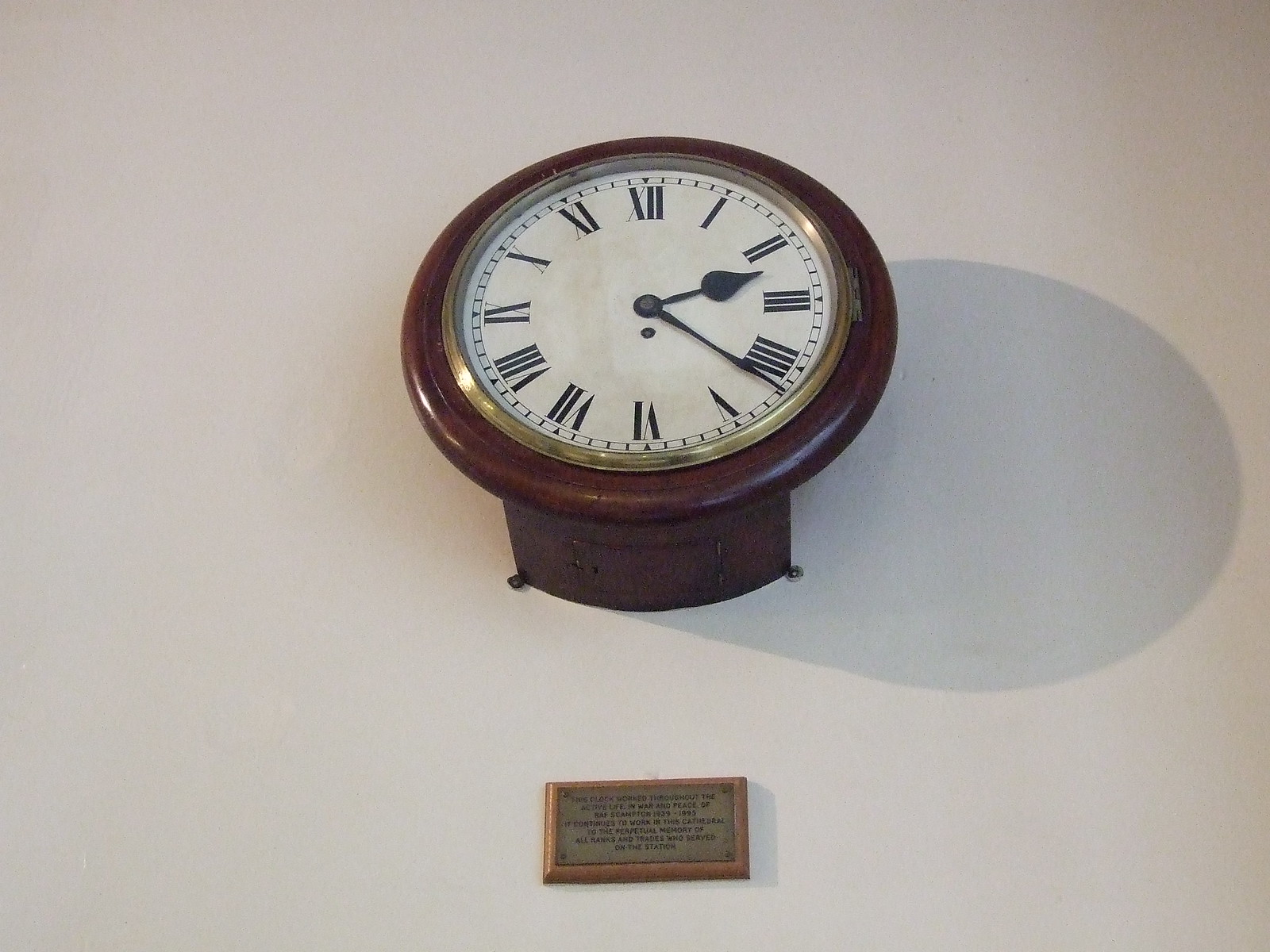This photograph showcases a distinctive round wooden wall clock. The clock is affixed to a grey wall and viewed slightly from below, revealing a dark wooden back mount that elevates it off the wall. The wooden clock features a white face encircled by a metal rim and a wooden border. Prominently displayed are Roman numerals and traditionally styled black clock hands, with the hour hand wider and teardrop-shaped while the minute hand is longer and skinnier. The time displayed is precisely 2:21. A notable small plaque lies just beneath the clock, consisting of a bronze or gold oblong metal piece set on a light wood base. While the plaque's text is unclear, it suggests the clock holds some form of significance, possibly commemorative. The clock casts a shadow to its right, adding depth to the scene against the otherwise plain grey wall.